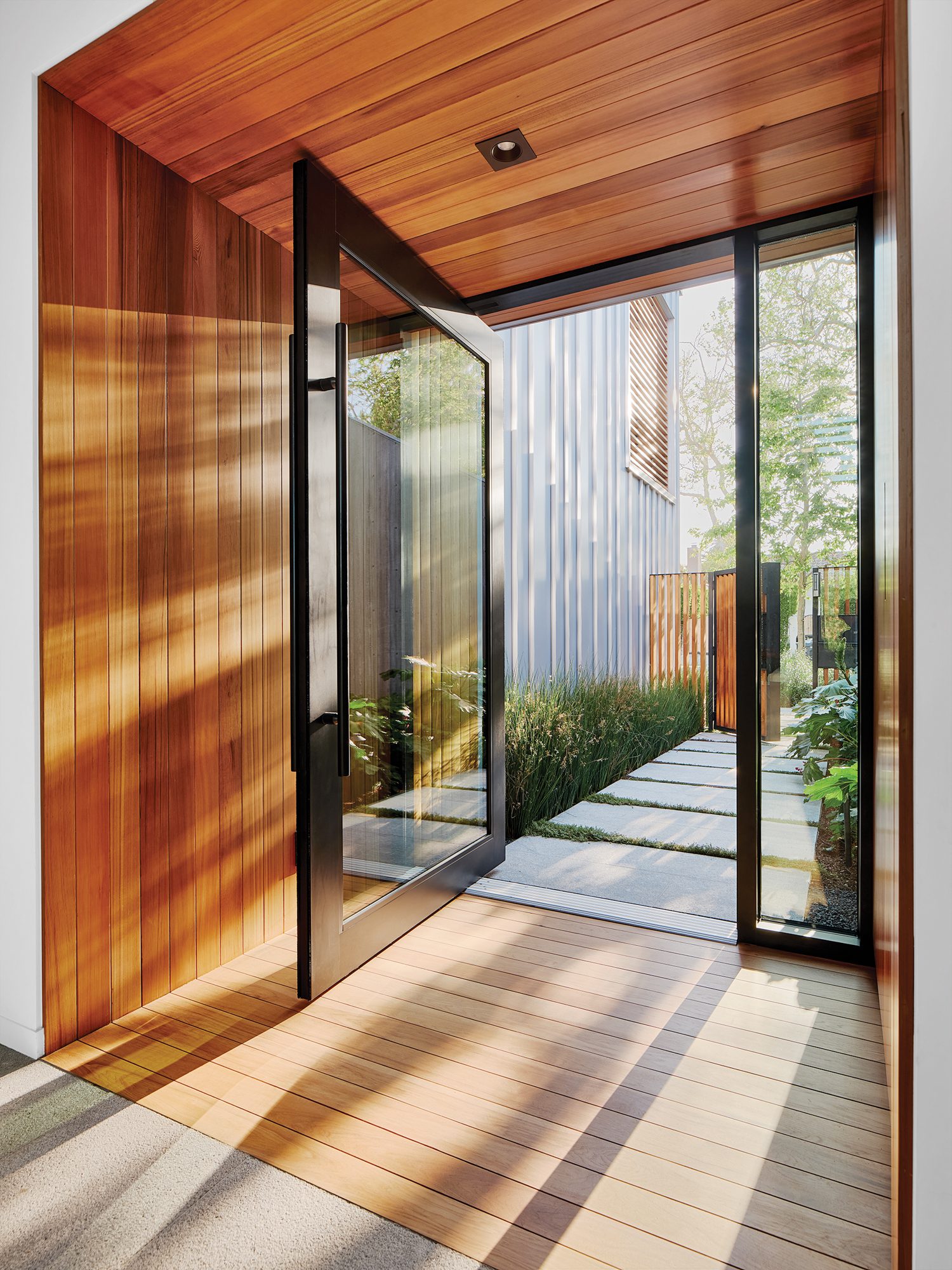The photograph captures the entryway of a luxurious, tall residential building. The entrance is dominated by a massive floor-to-ceiling glass door framed in dark material, with vertical handles that run the length of the door, reminiscent of those found in institutional settings. This grand doorway, which opens inward with inset hinges, is flanked on the right by another tall glass panel that stretches from floor to ceiling. The entryway is enveloped in rich, natural wood-stained planks that extend seamlessly across the floor, walls, and ceiling, lending a warm, cohesive aesthetic.

Inside, the home features pristine white walls and short tan-colored carpeting, a glimpse of which is visible on the bottom left of the photograph. Overhead, a small recessed LED light is set into a black square on the ceiling. Leading from the entryway to the exterior is a pathway composed of rectangular concrete stones. This path cuts through a surrounding of lush greenery, culminating at a wooden fence. Beyond the fence, trees can be seen, as well as a tall, shed-like structure on the left side of the fence, which complements the overall refined and naturalistic design of the residence.